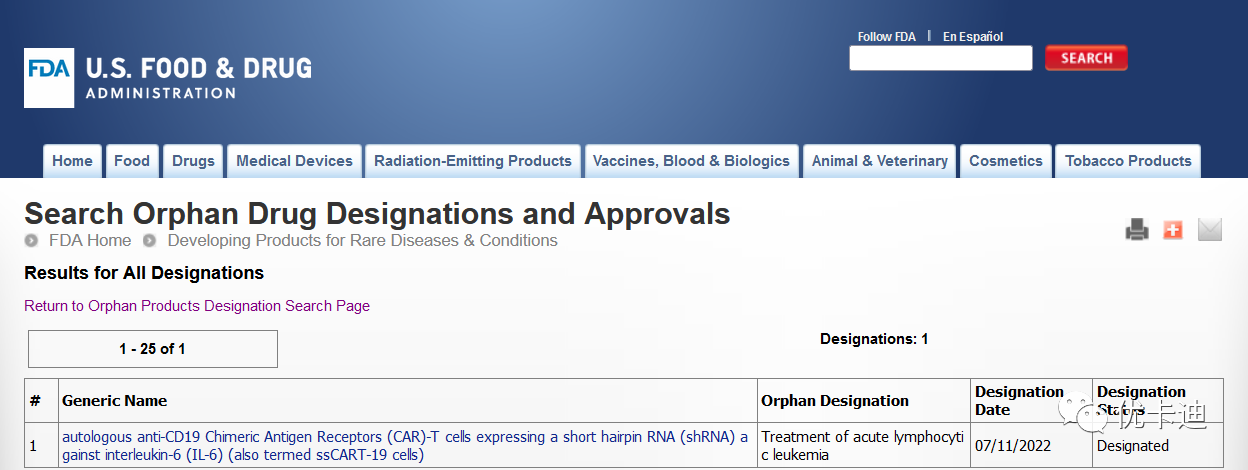The image features the official U.S. Food and Drug Administration (FDA) website interface. At the top of the page is a dark blue header with a prominent white square containing the FDA logo in blue. Below the header, the text "U.S. Food and Drug Administration" is displayed. A search bar, accompanied by a conspicuous red search button, is located beneath this text, with a note above it encouraging visitors to follow the FDA in Español.

Directly below the search bar, there are several navigational tabs in gray, labeled as follows: Home, Food, Drug, Medical Devices, Radiation-Emitting Products, Vaccine, Blood and Biologics, Animal and Veterinary, Cognitive and Tobacco Products. These tabs provide easy access to various sections of the FDA's website.

Further down, a large bold headline states "Search Orphan Drug Designation and Approvals." Directly underneath, in smaller text, links are provided for "FDA Home," "Developing Products for Rare Diseases and Conditions," "Results for All Designations," and "Return to Orphan Product Designation Search Page." The section details a generic name "Auto CD19," associated with Chimeric Antigen Receptors and T-cells in the context of short margin RNA.

The layout and detailed labeling of the website facilitate user navigation and highlight the FDA's role in overseeing the development and approval of treatments for rare diseases.